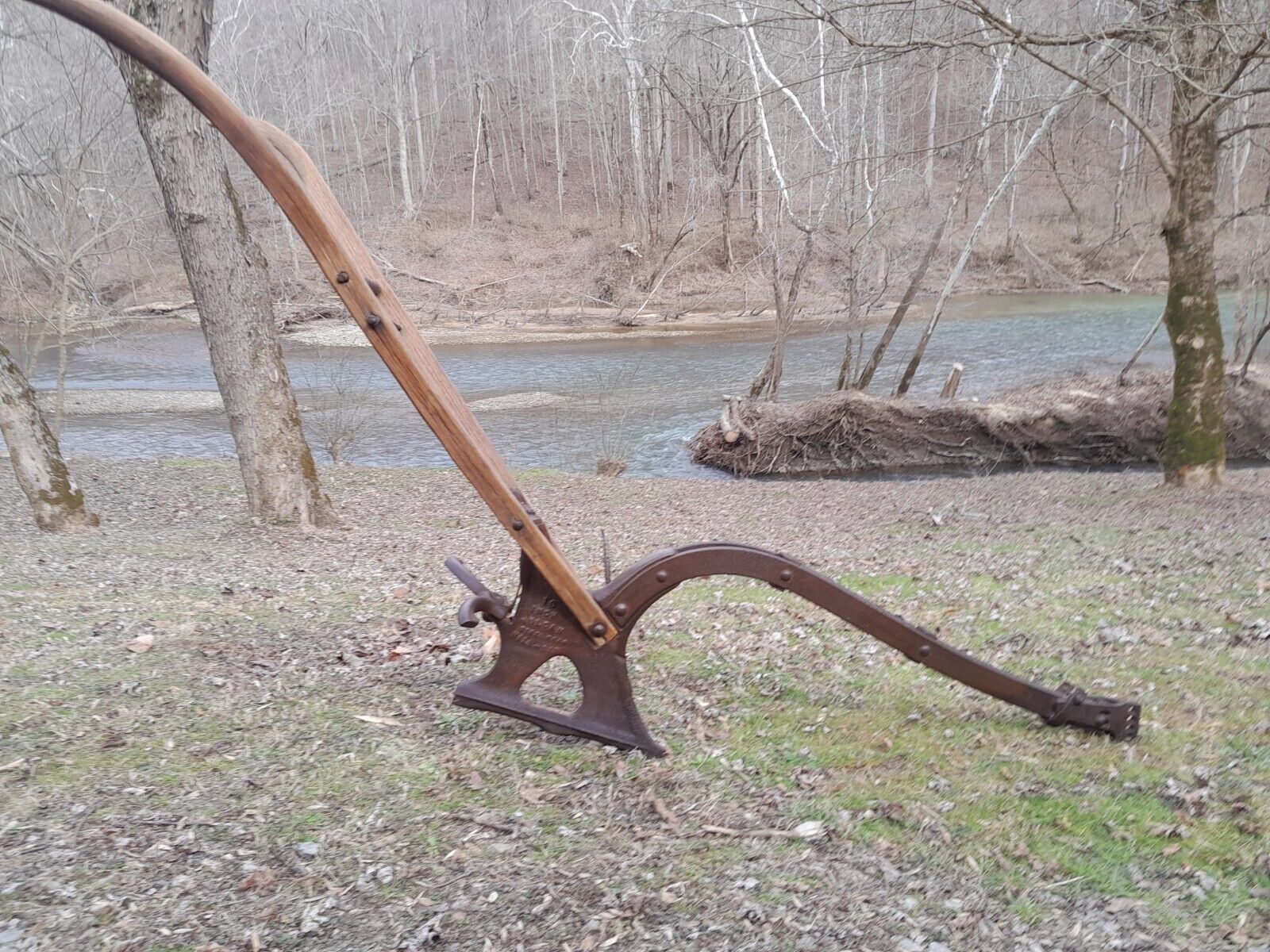The photograph captures a scenic outdoor landscape in fall or winter, featuring a diverse array of elements. In the background, a forest of bare, whitish-barked trees, possibly birch or aspen, lines the horizon. These trees stand behind a light blue and brown river, with a small sand bar near the right edge of the frame. This sand bar supports a few trees, their roots visible at the edge. The photo is set on a grassy area blanketed with dead leaves. The focal point in the foreground is a piece of industrial equipment, comprised of a large, curved metal base attached to a light brown wooden arm, partially cut off on one side of the image. Two trees flank the left upper corner and another tree stands on the right, completing this tranquil yet intriguing mechanical and natural tableau.